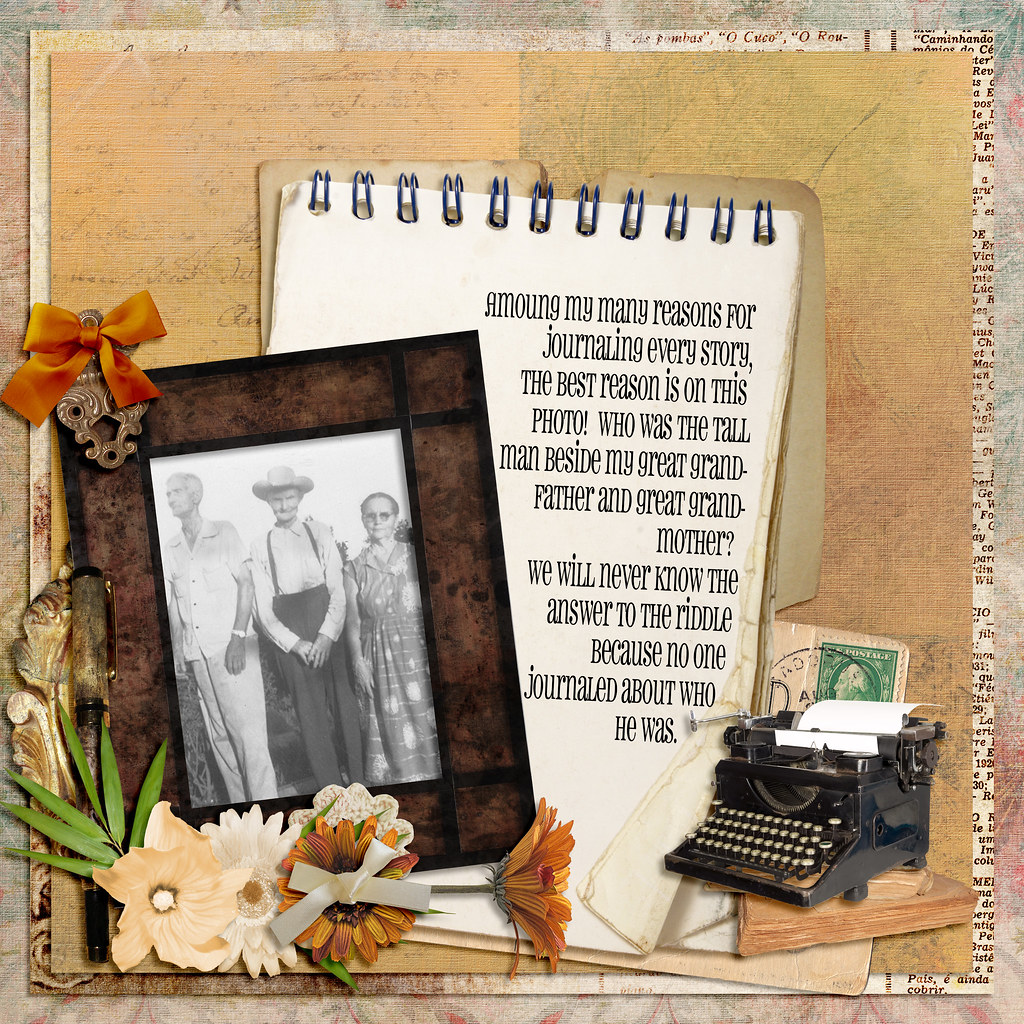The image features a meticulously crafted artistic slide with multiple layered borders. The outermost border mimics a canvas-like material adorned with a multi-colored floral pattern that acts as a frame. Inside, there's another inset frame made to resemble aged newspaper. Set against a textured, brown wallpaper-like background is a notepad with crisp white sheets. Within this notepad, in black text, is written: "Among my many reasons for journaling every story, the best reason is on this photo. Who was the tall man beside my great-grandfather and great-grandmother? We will never know the answer to the riddle because no one journaled about who he was."

In front of the notepad, centered on the left with a bow in the upper left corner, is a brown-framed, black-and-white photograph. The picture captures three individuals: a very tall man in white clothing with a watch on the left, a man in suspenders and a cowboy hat in the center, and a woman in a patterned dress and glasses on the right. The man in the center is identified as the speaker's great-grandfather, and the woman as the great-grandmother.

To the right of the notepad is a slightly smaller, vintage black typewriter with a piece of white paper in its roller. Additionally, a small ornate bow embellishes the photograph, and there are flowers positioned in the lower left-hand corner of the entire composition. Layers of elements, such as a fold at the bottom of the notepad and what appears to be a postage stamp, contribute to the intricate, scrapbook-like aesthetic of the image.